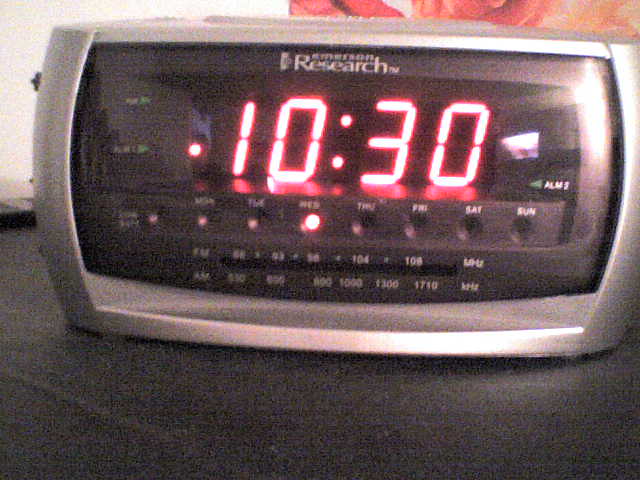This color photograph captures a close-up shot of a vintage-style rectangular clock radio. The clock radio features a grey metallic frame and a large LCD panel displaying the time, 10:30, in a white light with a reddish hue around the digits, creating a slightly blown-out effect. Below the display, there is a row of round buttons, and beneath them, additional buttons with white text labels beside each one. In the center of the device, there is a partially legible logo that reads “I Research.” The clock radio is placed on a dark black surface. The background reveals a greyish wall, with what appears to be a curtain adorned with a red or orange pattern towards the right side. Some glare is noticeable on the right and bottom edges of the clock radio. The overall image is grainy, exhibits poor quality, and is somewhat desaturated, lending a muted appearance to the scene.